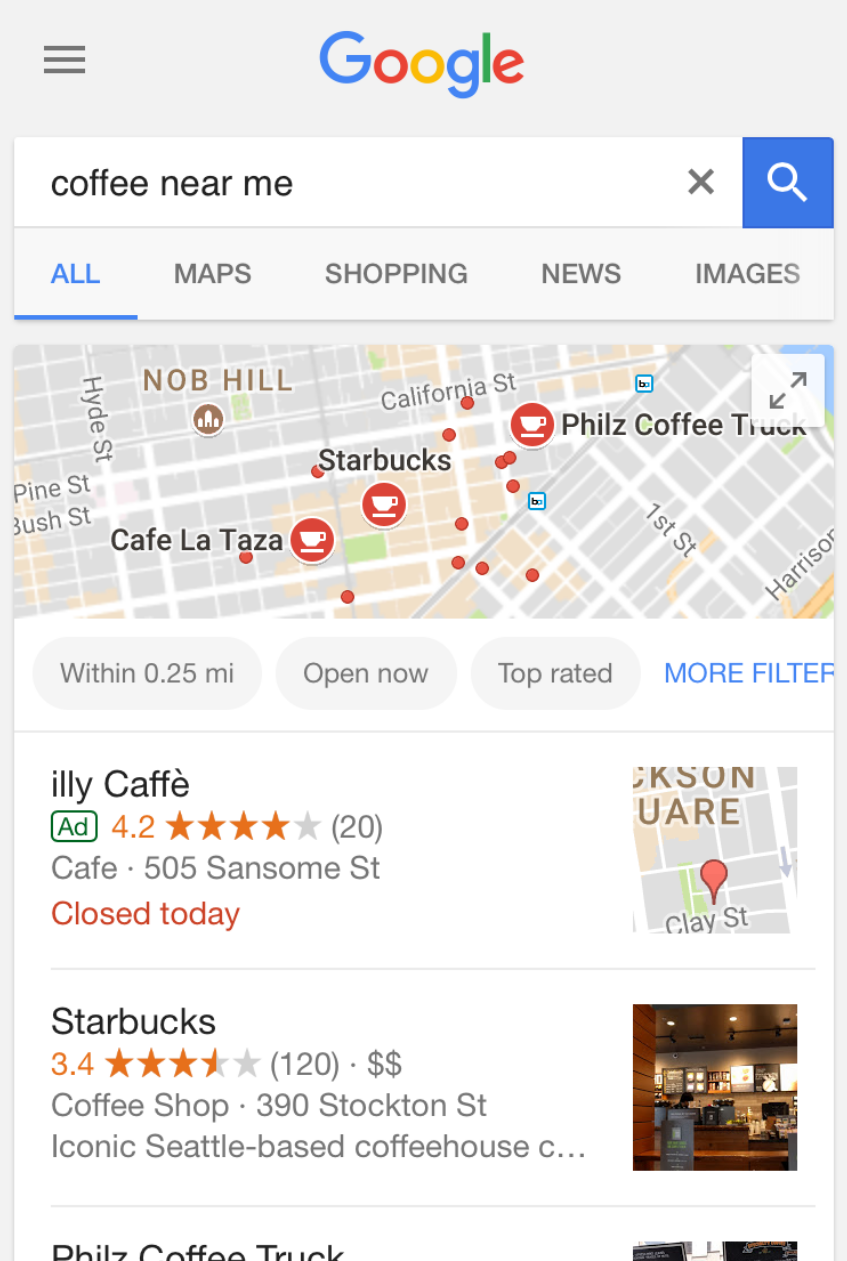Screenshot of a Google search on a mobile device showing results for "coffee near me" in portrait format. The Google logo is prominently displayed at the top, followed by a search bar where the query is typed in black. The search is currently set to the "All" tab, underlined in blue, with additional tabs including "Maps," "Shopping," "News," and "Images" in grey.

Beneath the search bar, a map displays various nearby coffee shops, marked with red circles outlined in white, each featuring a white coffee cup icon. Key places highlighted include "Philz Coffee Truck," "Starbucks," and "Cafe La Taza," all identified with bold black text. Additional smaller red dots signify other, possibly less popular or smaller coffee shops within the vicinity. 

Details indicate that the search results are filtered to display places "within 0.25 miles, open now, top rated." An ad for "Ili Cafe" appears below the map, noting it is "closed today," with an option to view its location on the map, although it isn't marked by name.